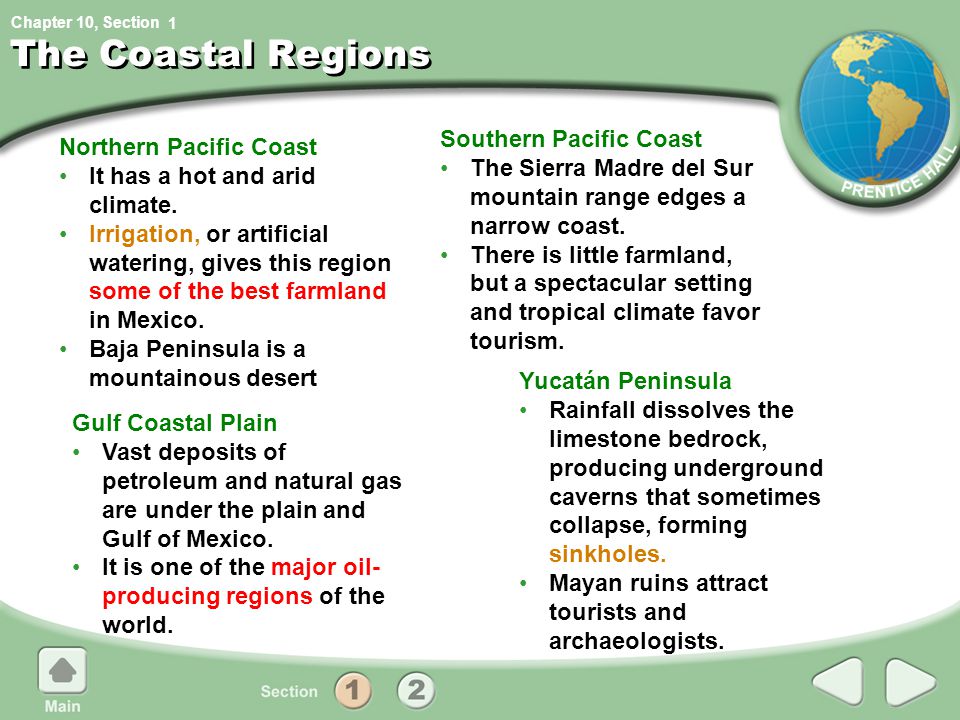A detailed interactive computer slide about the coastal regions from Chapter 10, Section 1: "The Coastal Regions," with a light green header and footer. The top left features small text indicating the chapter and section, while the title "THE COASTAL REGIONS" is prominently displayed in larger white capital letters. On the right side, a small image of a globe is labeled "Prentice Hall."

The central part of the slide, set against a white background, details various coastal regions with color-coded text. Firstly, the **Northern Pacific Coast** is highlighted in green, noting its hot and arid climate, and the importance of irrigation (in yellow) for creating some of Mexico's best farmland (in red). Next, the **Baja Peninsula** is described as a non-mountainous desert.

Below, the **Gulf Coastal Plain** is introduced in green text, mentioning vast deposits of petroleum and natural gas under the plain, making it one of the world's major oil-producing regions (with "major" emphasized in red).

To the right, the **Southern Pacific Coast** is outlined in green text, focusing on the Sierra Madre-Del Sur mountain range edging the narrow coast. Although there is little farmland, the spectacular setting and tropical climate are favorable for tourism.

Lastly, the **Yucatan Peninsula** section, also in green, describes how rainfall dissolves the limestone bedrock, creating underground caverns that may collapse to form sinkholes (highlighted in yellow). The Mayan ruins here attract tourists and archaeologists.

The bottom left corner features a home button for returning to the main screen, the center bottom has "Section 1, 2" for navigation, and the bottom right includes arrows for navigating forward and backward through the slides.